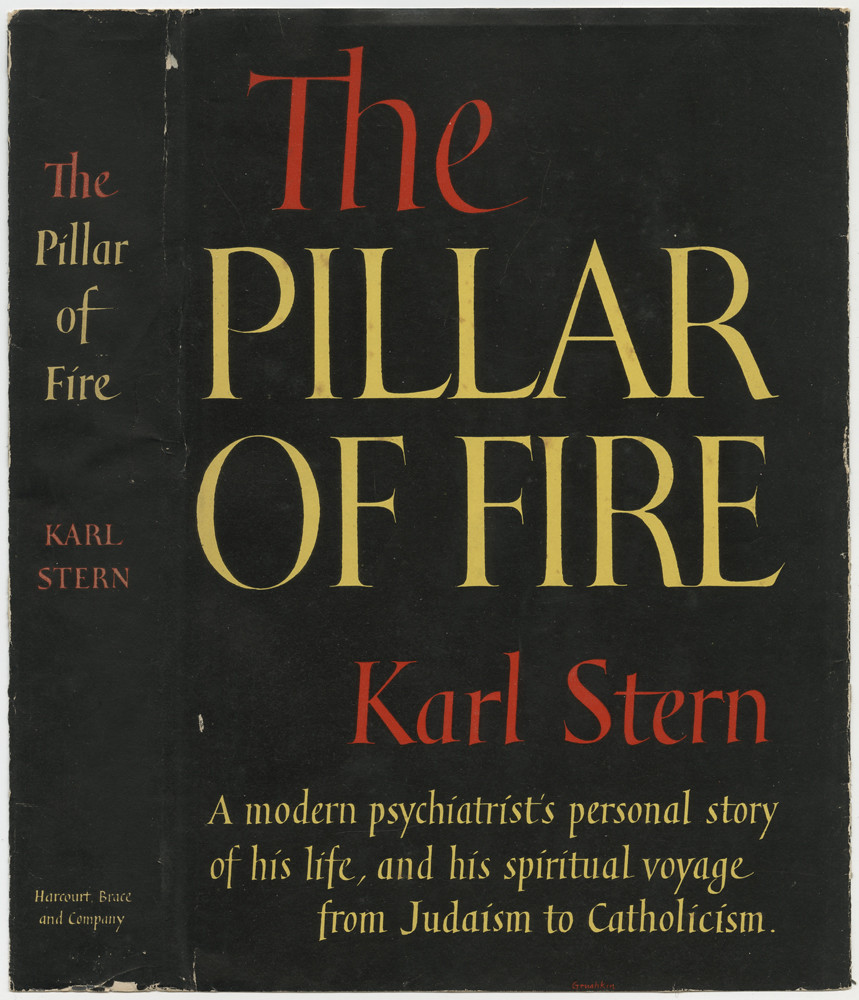The image depicts both the spine and the front cover of a novel titled "The Pillar of Fire" by Carl Stern. The cover and spine feature a basic black background with the title and author’s name prominently displayed. The title, "The Pillar of Fire," is arranged across multiple lines, with "The" and "Carl Stern" in red text and "Pillar of Fire" in yellow. Below the author’s name on the front cover, it reads, "A Modern Psychiatrist's Personal Story of His Life and His Spiritual Voyage from Judaism to Catholicism," in yellow, slightly gold-shaded text. The spine of the book also displays the title and author's name in similar fashion, with sufficient horizontal spacing. Additionally, the spine notes that the book is published by Harcourt Brace and Company. The cover is devoid of illustrations, featuring only the text, with some minor white elements indicating where the black has chipped away. The overall design uses a font that appears slightly script-like and traditional.